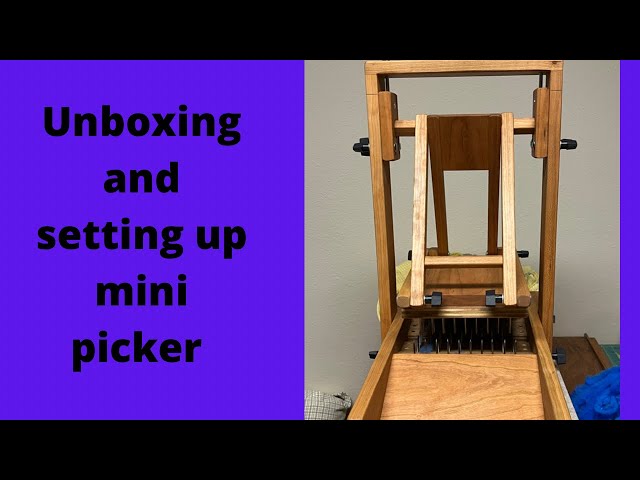The image displays a device called a "mini picker" against a purple background with a very basic border. The text "Unboxing and Setting Up Mini Picker" is prominently displayed within this border. To the right of the image, on a counter, sits the mini picker—a wooden contraption that somewhat resembles a catapult, featuring prongs in front and a trellis-like structure. Handles are present on the sides, and a piece of wood in the middle has a square cut out. Adjacent to the device, there is a blue cloth on the floor and a bag next to it. The function of the mini picker is unclear, but it appears to have knobs and blades, possibly designed to process or pick items by rolling them down a ramp.